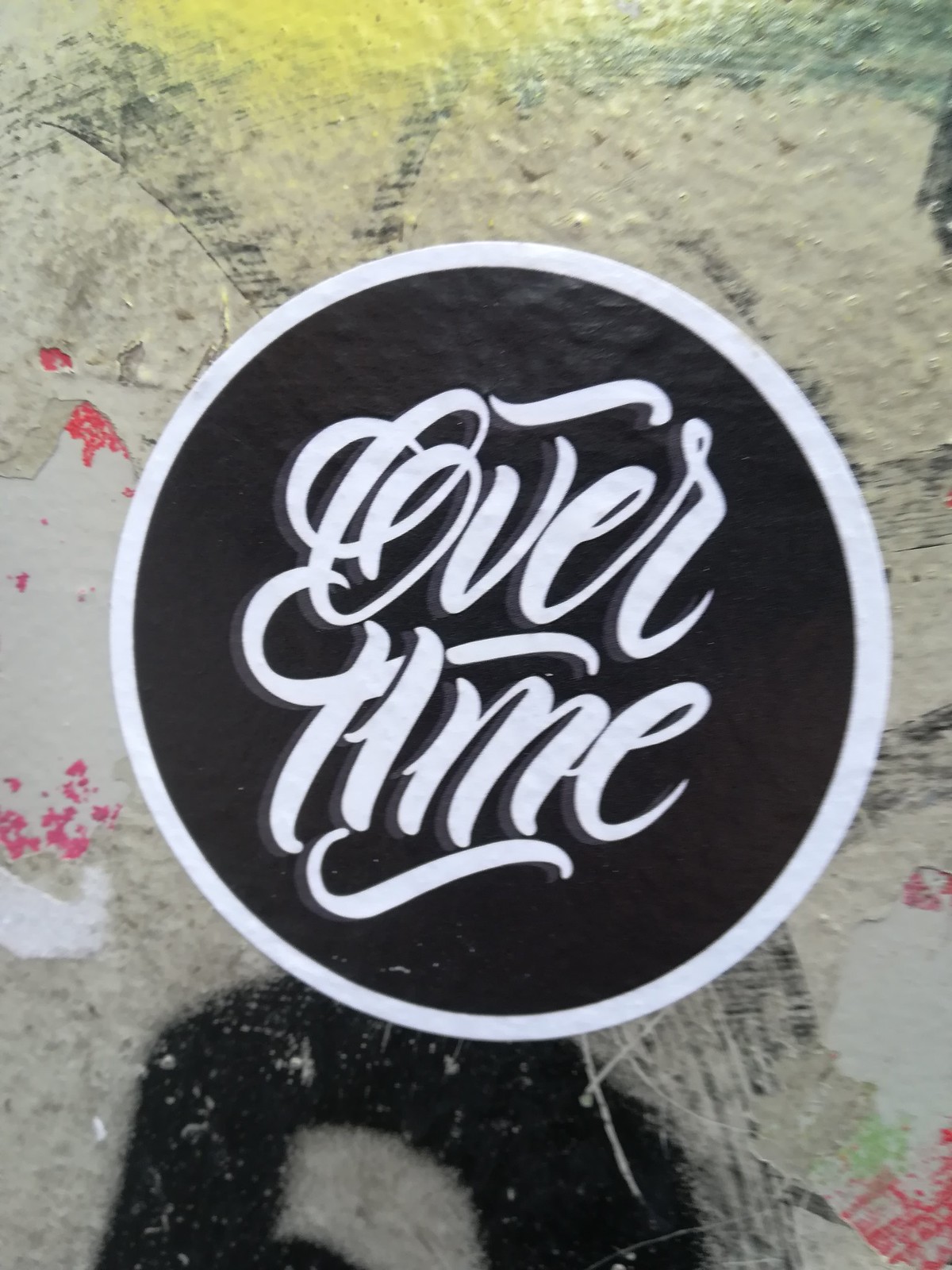This is a highly detailed close-up photograph of a round sticker or label affixed to a wall. The central feature is the sticker, which reads "Over Time" in elaborately styled, white cursive letters against a solid black background. The sticker itself is delineated by a white circular border. The wall behind the sticker serves as a colorful and visually stimulating backdrop. This background comprises an olive hue with splashes of green, red, and yellow paint. Additionally, there are smears of black and pink paint, with the pink primarily located at the lower right and center left sections. The wall also features stylized graffiti, including what appears to be a black-and-white image of a person's face, suggesting black hair, a white forehead, and dark eyebrows at the bottom center of the design. Overall, the composition of the image suggests a deliberate artistic effect, with the contrasting colors and patterns contributing to a striking visual impact.